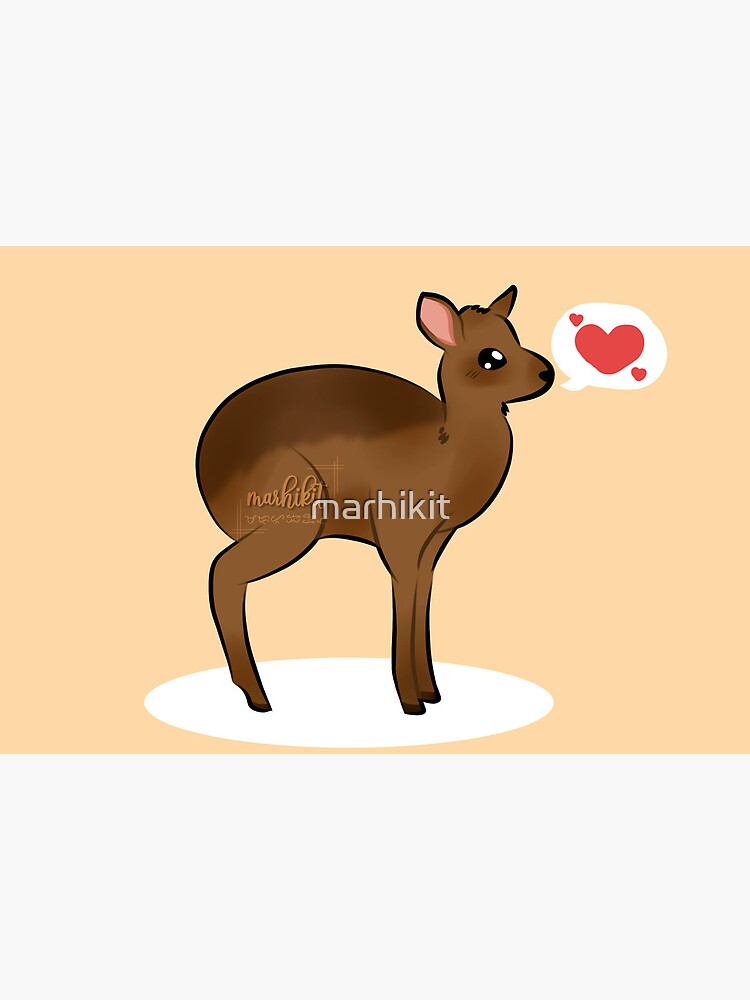This digital drawing showcases a cartoonish baby deer or fawn, predominantly brown with a slightly darker hue on its back. The fawn, facing right, is characterized by large black eyes with light reflections, pink ears, and is depicted standing in the center of a white oval against a peach-colored background. Emerging from its mouth is a speech bubble containing a large red heart flanked by two smaller red hearts. The image, set in a portrait orientation but framed by thick light gray borders giving it a landscape feel, features the semi-transparent watermark "Mar Hakit" across the center and the artist's handwritten signature "Mar Hickett" to its left.